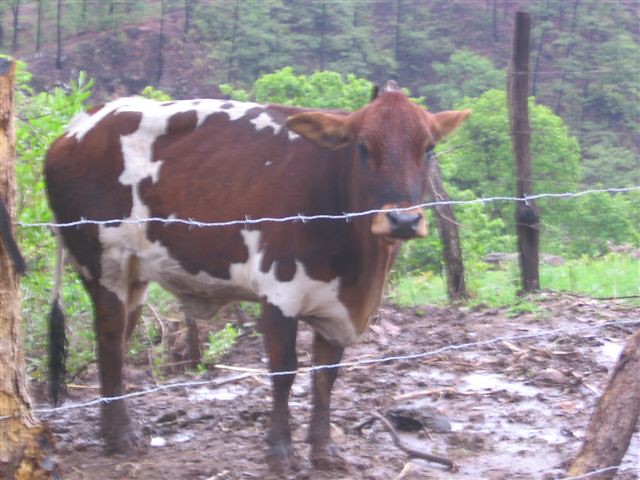In this image, a predominantly brown cow with white patches along its back and underbelly stands in a muddy and wet enclosure. Its face, legs, and rump are entirely brown, and its noticeable white markings include a line running along the spine. The cow is enclosed by a simple wire fence supported by wooden posts on either side. The backdrop features lush greenery with an abundance of green leaves and tree trunks, indicating a wooded area on a sloped hillside. The enclosure may also extend further back, as more wooden poles are visible before the line of trees. The cow, with a black nose and alert ears, is looking directly at the camera, adding a touch of personality to the scene.